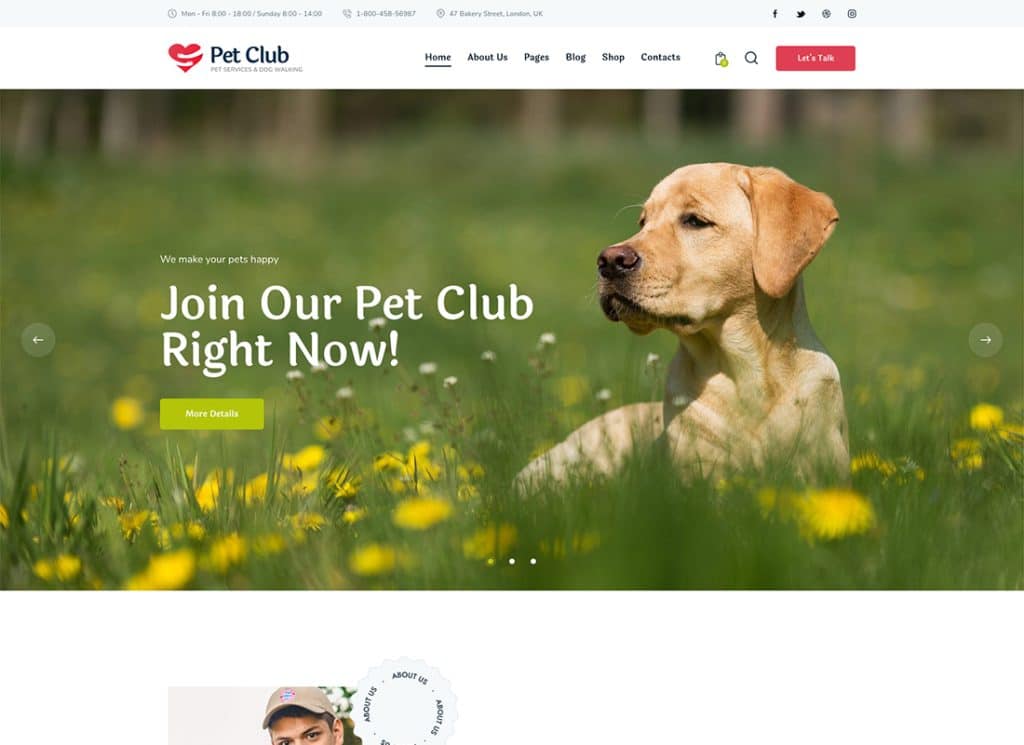The screenshot captures a vibrant and well-organized website for a pet care service named "Pet Club." In the header, there is a prominent logo featuring a red heart being embraced by white arms, symbolizing care and affection. Positioned at the top of the page, there are contact details including a phone number and an address in the U.K. Navigation is user-friendly, with a menu listing sections like Home, About Us, Pages, Blog, Shop, and Contacts. 

Adjacent to the navigation menu, there are icons for social media platforms, ensuring easy connectivity. A magnifying glass symbol indicates a search function, and beside it, a clipboard icon displays notifications or updates. Prominently, there is a red button labeled "Let's Talk" to facilitate quick communication.

Dominating the center of the page is a captivating image of a tan-beige dog looking leftward, exuding a sense of peaceful contentment. Superimposed on this picture is the slogan "We Make Your Pets Happy" in small print, complemented by a bold, inviting message "Join Our Pet Club Right Now." Below this call-to-action is a green clickable box offering "More Details" for prospective clients.

The cohesive design and thoughtful elements of this website underscore the dedication to providing comprehensive pet services, from dog walking to a variety of pet care solutions.